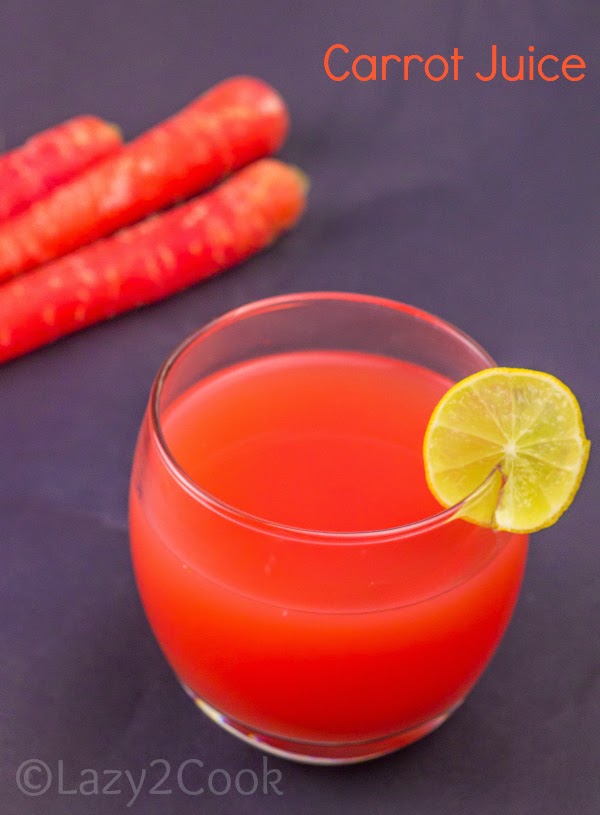The image features a small, transparent tumbler filled almost to the top with deep orange carrot juice, which is the focal point of the composition. The tumbler is positioned in the lower right corner, occupying about half of the image. A yellow-tinged lemon wedge adorns the rim of the glass. Encircling the glass is a dark purple or perhaps very dark fabric background. On the left side of the image, slightly out of focus, there are three bright orange carrots. At the top right corner, the words "carrot juice" are written in a thin bright orangey-red font. Lastly, in the bottom left corner, a pale purple watermark reads "© Lazy 2 cook" as one word.